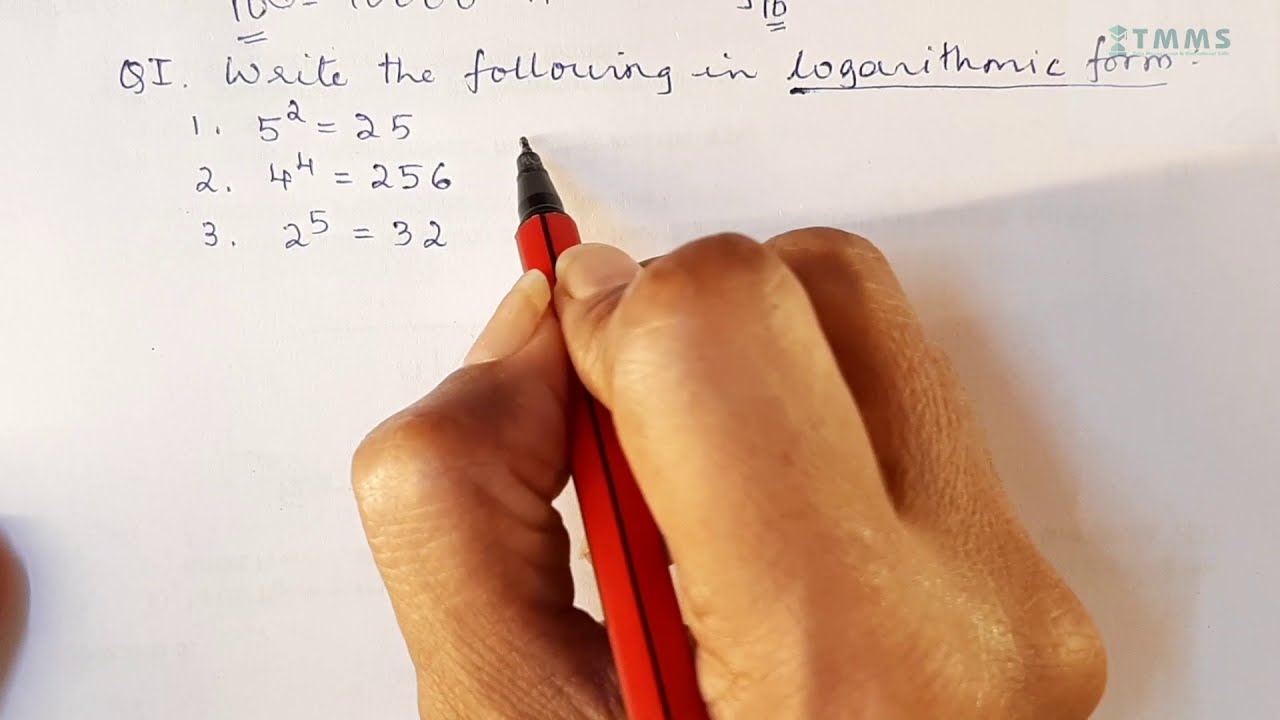The image is a close-up of a white sheet of paper, centered around a right hand holding a red pen with a black stripe and a black tip. The pen is writing in blue ink. The hand, extending from the bottom of the image, is depicted from the knuckles to the fingertips, with the thumb positioned to the left and fingers to the right. The light source is coming from the left, casting a shadow to the right of the hand. The text on the paper reads: "Q1. Write the following in logarithmic form," with "logarithmic form" underlined. Underneath, three mathematical expressions are listed: "1. 5² = 25," "2. 4⁴ = 256," and "3. 2⁵ = 32." The image captures the hand as it is in the process of writing, suggesting more text might follow.